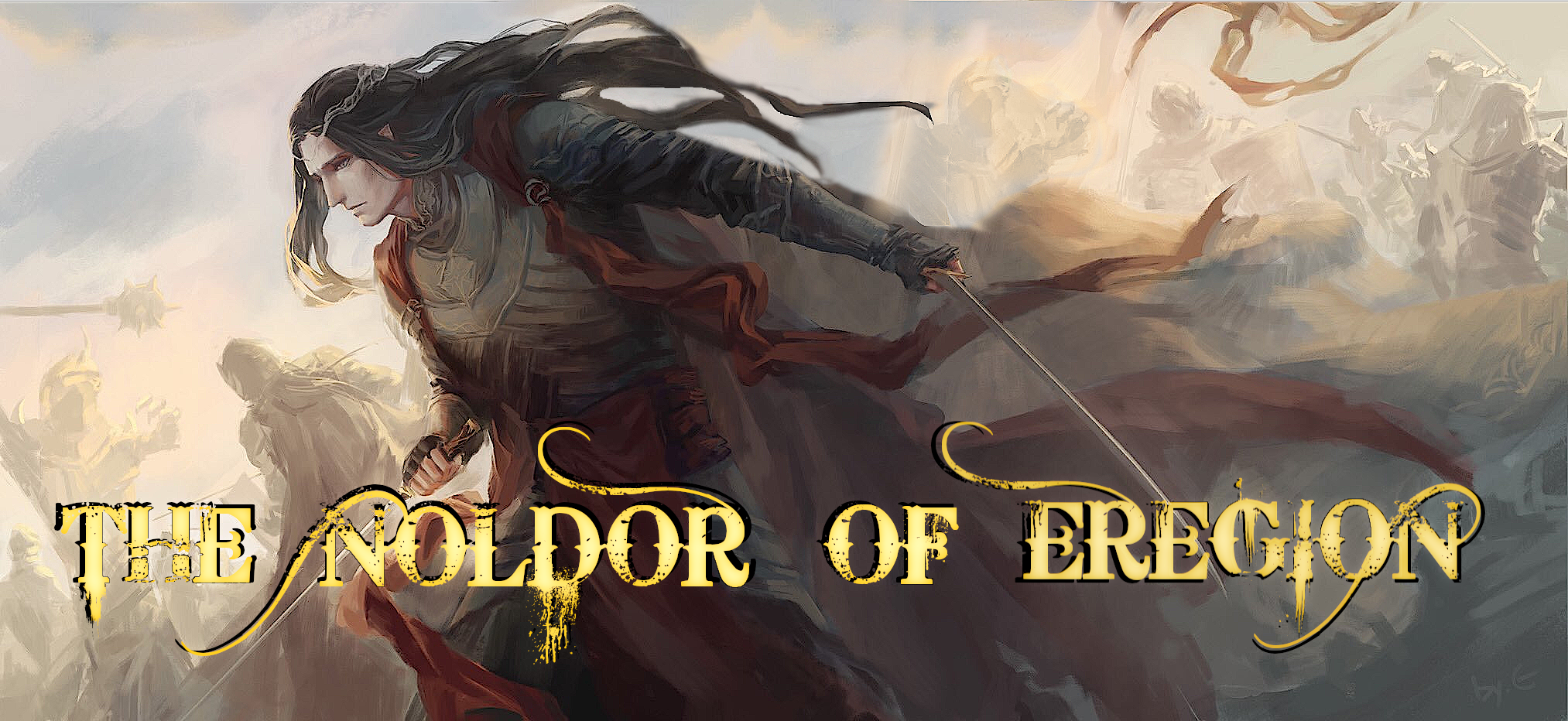This image appears to be an elaborate drawing, possibly a promotional poster for a video game, movie, or story titled "The Noldor of Eregion." Central to the image is a striking elf-like figure with long black hair and very white skin, donned in black leather armor adorned with red sashes. This intense character wields a long knife in both hands, standing out vividly in color against the more subdued, whitish-gray tones of the background. The background itself depicts a chaotic battle scene with numerous warriors engaged in combat, one wielding a spiked mace. Despite the lack of clarity about who is fighting whom, the detailed depiction of this main figure, with flowing hair and gold-embellished attire, draws immediate attention. The caption "The Noldor of Eregion" is elegantly written at the bottom in a fancy golden font, further adding to the poster's intricate and captivating design.